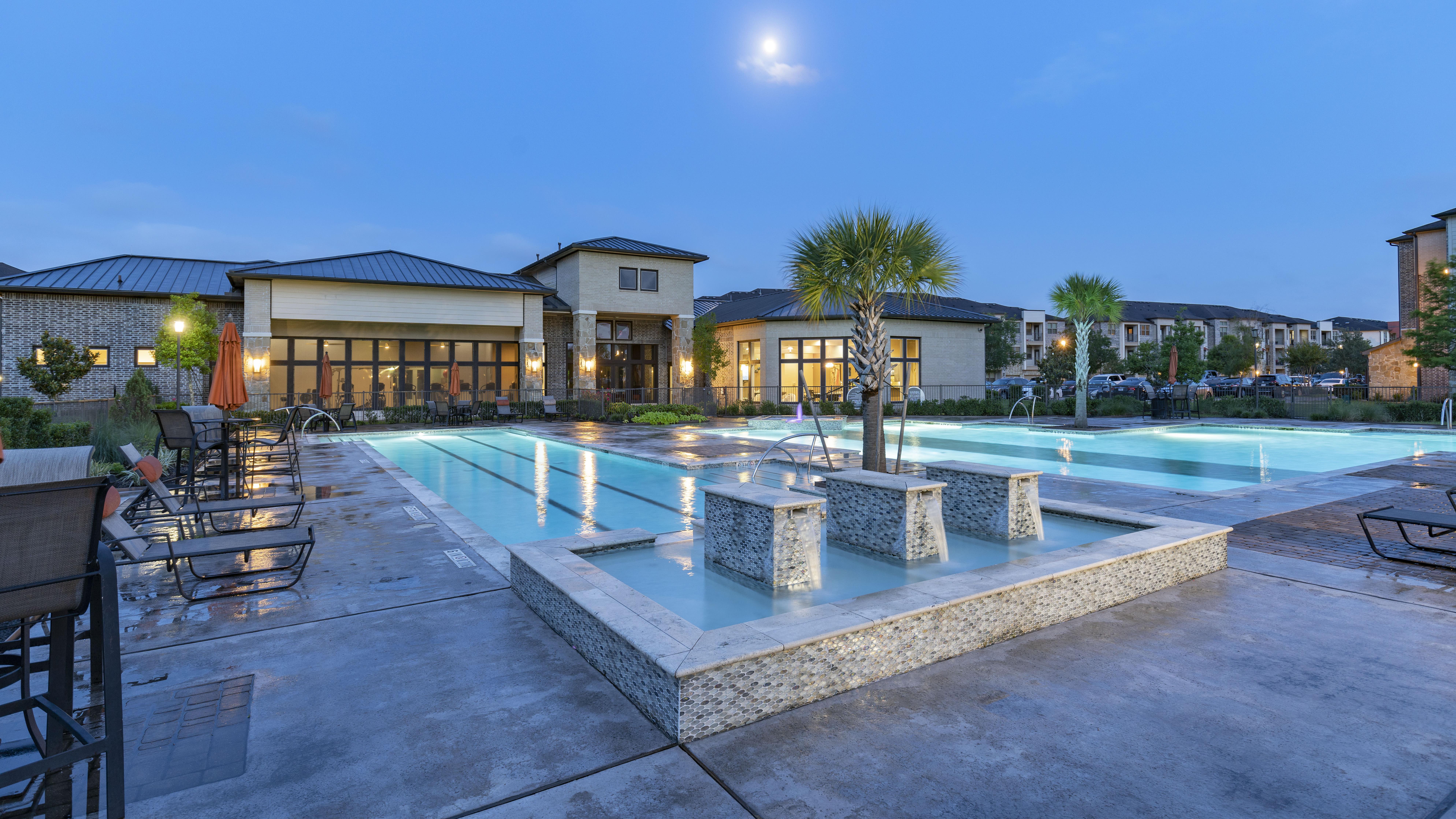This image depicts an elaborate evening scene at an outdoor courtyard featuring an interconnected series of three illuminated swimming pools, characterized by their bright blue water and underwater lights. Surrounding the pools is a broad concrete plaza equipped with numerous lounge chairs and tables, suggesting areas for relaxation and gatherings. The scene also incorporates landscaping elements, including concrete islands with palm trees and shrubs adjacent to the buildings.

In the background, a row of one-story structures with expansive glass windows, likely public meeting spaces, is prominent. They are well-lit and bustling with numerous people inside. To the right, a towering multi-storied building, potentially a hotel or apartment complex complete with parking facilities, rises against the night sky. The visible moon hints at the late hour, casting a dark yet serene ambiance over the setting.